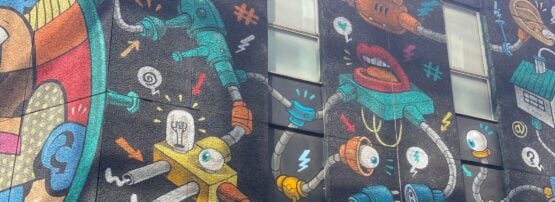This photograph showcases a close-up view of the side of a black-painted building adorned with a highly detailed and abstract mural. Central to the mural are cartoonish depictions of various technological elements intertwined with human features, predominantly themed around eyeballs and lips. A prominent feature is a blue platform with red lips, teeth, and a tongue, connected by various cables and silver piping extending throughout the mural. To the left, another platform exhibits a large light bulb paired with blue, white eyeballs. The mural also includes surreal, mechanical apparatuses in shades of turquoise and teal, with arrows, blue lightning bolts, orange hashtags, and thought bubbles that contain hearts and swirls. The mural’s intricate designs surround two beige-shaded, rectangular windows, framing a vividly imaginative scene where machinery and whimsical elements blend seamlessly.